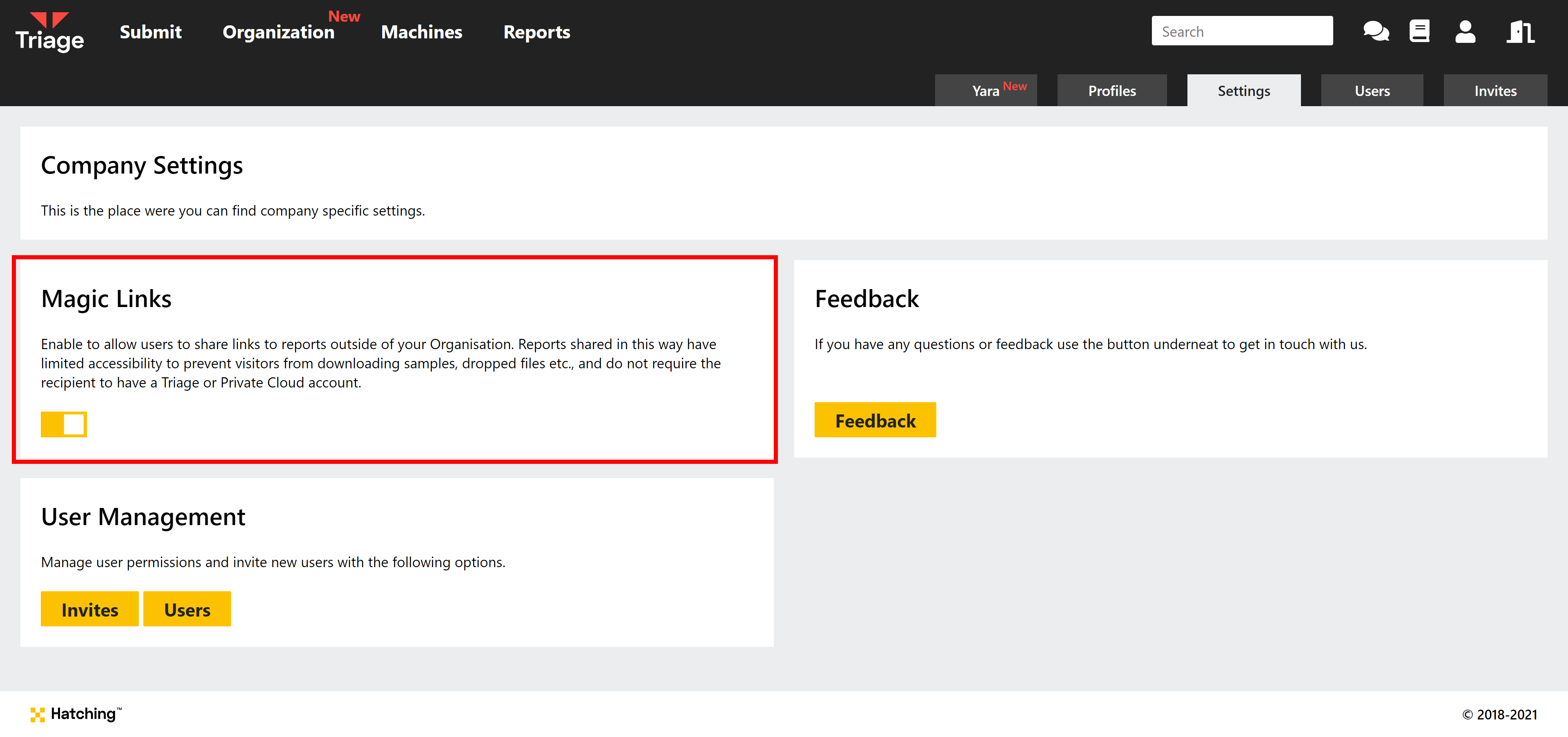This horizontally oriented image is a screenshot from a website, accessible via computer or smart device. At the top is a long, dull black rectangular strip. In the upper left corner, there's a small triangle icon labeled "Triage" in white, accompanied by options "Submit" and "Organization." Above these, "New" is highlighted in red, followed by "Machines" and "Reports."

To the right, a search bar is present alongside various clickable white icons. Below this, several gray rectangular boxes with white lettering can be seen. They include "Yara" marked with "New" in red, "Profile Settings" (currently selected in white), "Users," and "Invites."

Proceeding downward, a white box displays "Company Settings" in black, indicating where to find company-specific configurations. Below this, "Magic Links" is written in black, followed by a brief description, all enclosed within a red-bordered box. A yellow progress bar, half-filled, divides this section.

Underneath, another white rectangular box is labeled "User Management" in black, explaining how to manage user permissions and send new invitations with options like "Invites" or "Users." Lastly, a feedback section offers assistance, stating, "If you have any questions or feedback, use the button underneath to get in touch with us." A yellow box with black lettering reads "Feedback."